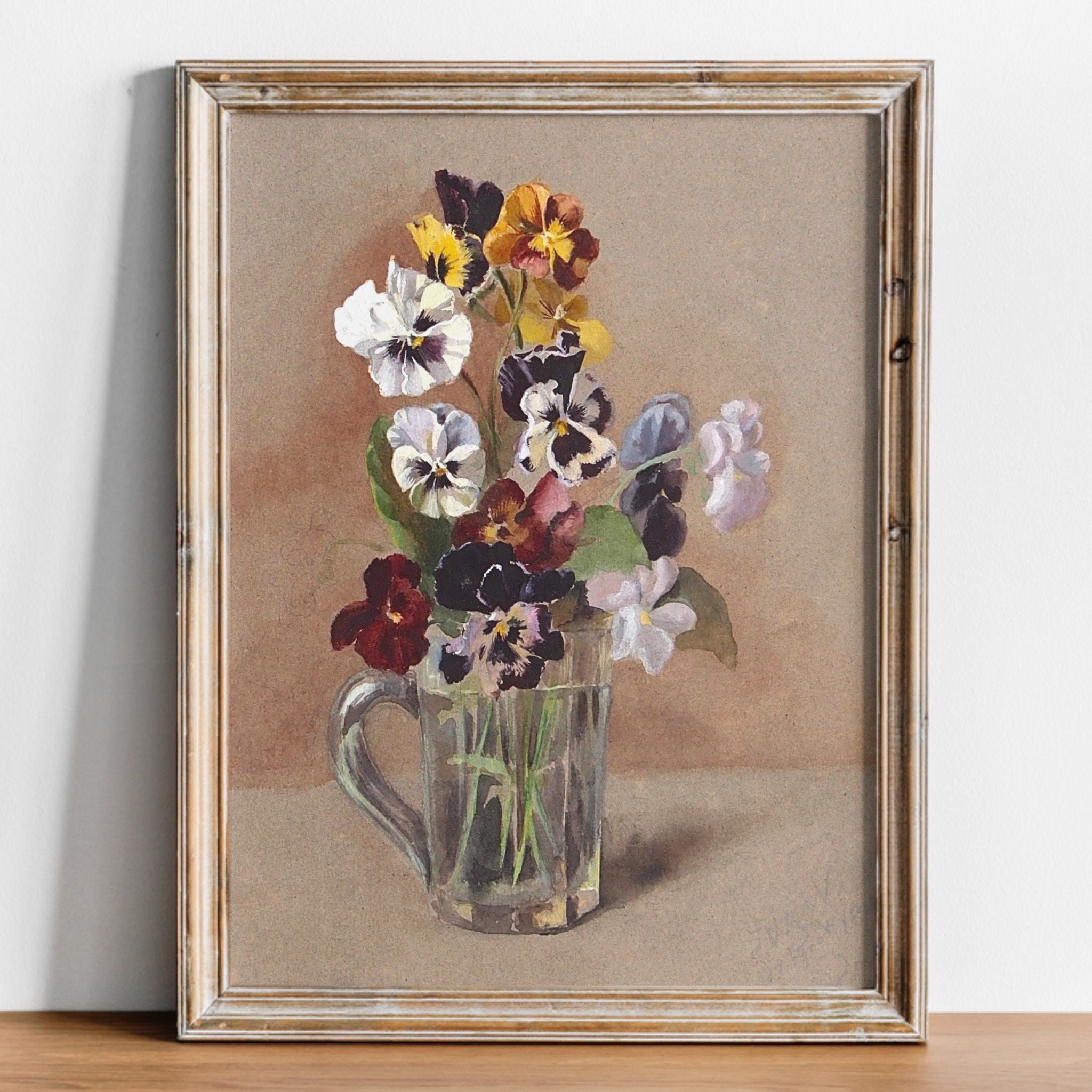In the image, there is a detailed painting depicted inside a wooden frame, featuring visible knots on the right and top edges. The painting is leaning against a pristine white wall on a rich brown wooden floor. The background of the painting has a grayish-tan hue, and it portrays a still life scene with a glass pitcher, nearly filled with water, resting at the bottom center. The water inside the pitcher clearly shows the stems of the flowers it holds. The bouquet within the pitcher includes a vibrant mix of flowers: maroon, white, lavender, with prominent yellow and orange hues at the top. Additional details include flowers with various centers—white with a purple center, red with a yellow center, and dark blue with pink, blue, and yellow centers. Surrounding the flowers are a few leaves adding to the natural beauty of the arrangement. The frame itself gleams with a gold-like color in a beveled style, enhancing the elegance of this still life watercolor painting.